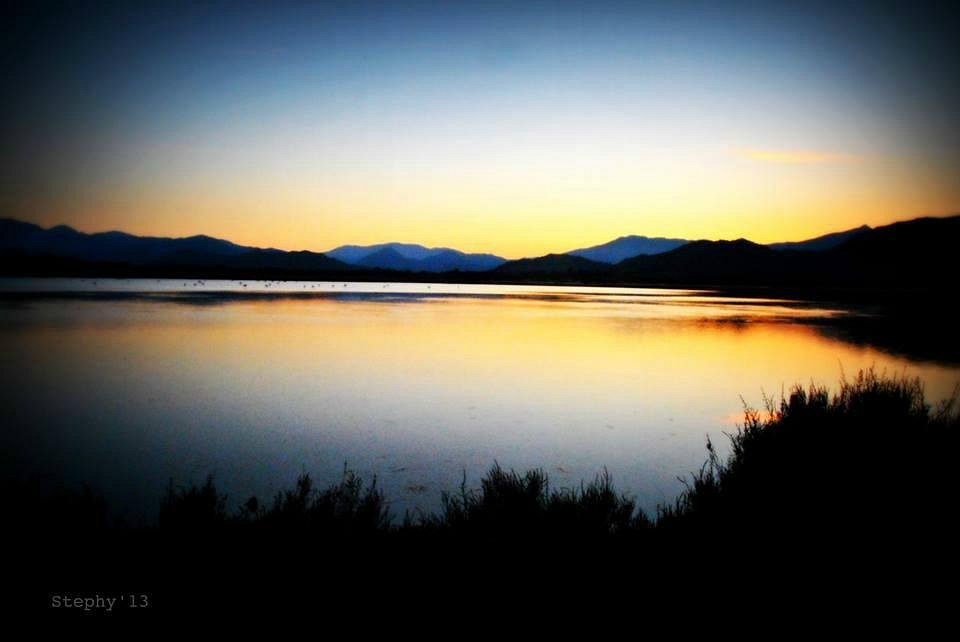An evocative photograph capturing an evening scene at a serene lake, illuminated by the warm hues of a setting sun. The sky transitions from a deep blue at the top to lighter shades of orange and yellow near the horizon, painting a picturesque backdrop reflected beautifully on the calm water of the lake. Gentle ripples disturb the lake’s surface, which mirrors the sky and distant mountains perfectly, creating a captivating reflection. Silhouettes of short grass and bushes frame the foreground, adding depth to the image, while tiny specks, likely distant birds, dot the water. The edges of the photograph fade to black, enhancing the central glow. Notably, the bottom left corner of the image bears the signature "Steffi '13," indicating the artist's name and perhaps the year the photo was taken.